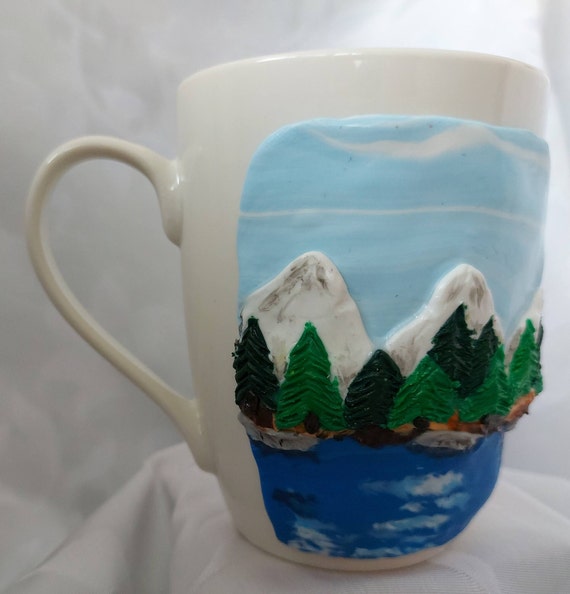The image showcases a custom-made, white ceramic coffee mug with intricate, textured artwork on its front. The artwork, which appears to be hand-sculpted from clay and then attached to the mug, forms a roughly rectangular panel. This panel features a vividly detailed landscape scene: at the bottom, there's a blue body of water with white ripples, possibly indicating a lake or river. Adjacent to the water are rocks and a line of pine trees in varying shades of green, some light and others dark. Rising behind the trees are snow-capped white mountains, and above them, a pale blue sky adorned with streaks of white clouds. The mug itself rests on a white tablecloth, which also serves as the background, with a light gray hue visible in the upper part of the image. The handle of the mug, positioned on the left side, further emphasizes the mug's functional yet artistic design.